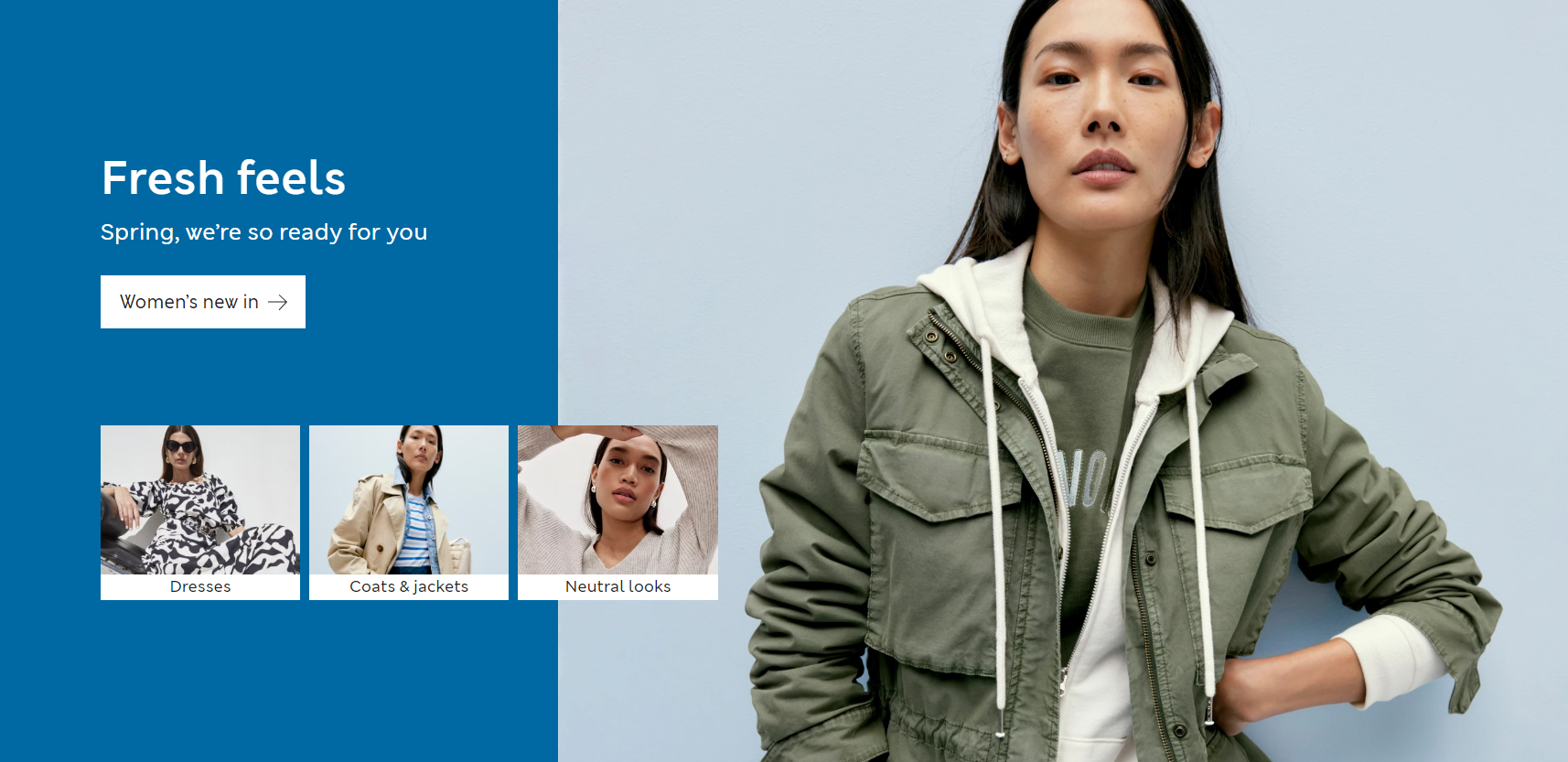This advertisement image, likely from a website homepage or an email campaign, is laid out in a left-to-right horizontal format. On the left side, a vertical cerulean blue box features the bold white text "Fresh Feels," followed by the less bold text "Spring, we're so ready for you." Below this, a white box contains the black text "Women's New In," accompanied by a clickable arrow for more options. Adjacent to this, there are images of a woman showcasing various outfits categorized under "Dresses," "Coats and Jackets," and "Neutral Looks," each with clickable links for further exploration.

The right side of the image transitions to a lighter grayish-slate blue background, highlighting a woman who appears to be Asian. She has long hair and wears an army-green sweatshirt emblazoned with partially obscured letters, over which she dons an army-green jacket and a white zip-up coat. Her hand is confidently placed on her hip as she gazes directly at the camera, conveying a sense of poise and readiness for the new fashion season.